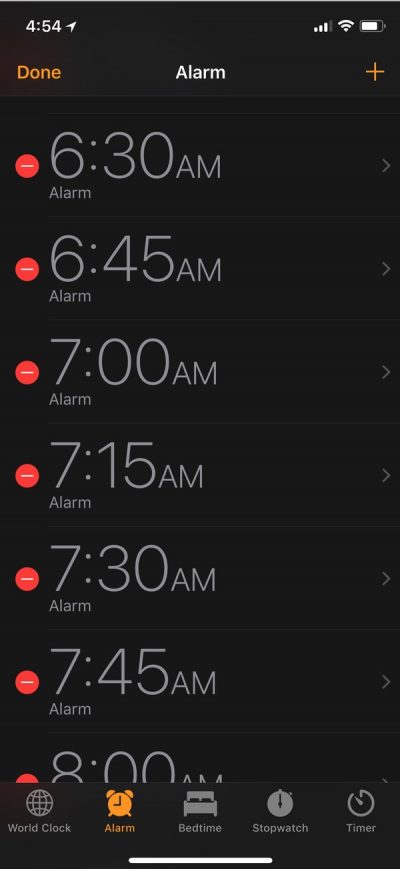The image is a vertical screenshot resembling the alarm interface of a smartphone, likely an iPhone or Android, with a predominantly black background. 

In the top left corner, "454" appears in white text, accompanied by an arrow pointing to the upper right. To the far right, the standard status icons are visible: a signal strength indicator showing three out of four bars, a Wi-Fi symbol, and a battery icon indicating approximately 75% charge. Below the "454," in the middle-right, the word "DONE" is displayed in orange letters.

Further down, in the same row on the far right, "ALARM" is written in white letters next to an orange plus sign. Following that, there's a vertical list of red circles, each containing a white horizontal slash. These red circles are aligned to the left of various alarm times. The listed times, each followed by the word "ALARM" in gray text, are as follows: 

- 6:00 AM
- 6:30 AM
- 6:45 AM
- 7:00 AM
- 7:15 AM
- 7:30 AM
- 7:45 AM
- 8:00 AM (partially cut off)

To the far right of each time entry, a sideways-facing gray "V" is displayed.

At the bottom of the screen, a menu of clickable icons is present:

1. A globe icon labeled "WORLD CLOCK" in gray.
2. An orange alarm clock icon, indicating the active Alarm page, with the word "ALARM" underneath.
3. A bed icon labeled "BEDTIME" in gray.
4. A stopwatch icon labeled "STOPWATCH" in gray.
5. A half-circle icon with an hour hand pointing to the upper left, labeled "TIMER" in gray.

A long white bar runs along the very bottom of the interface, completing the layout of what appears to be the ALARM page on a smartphone.